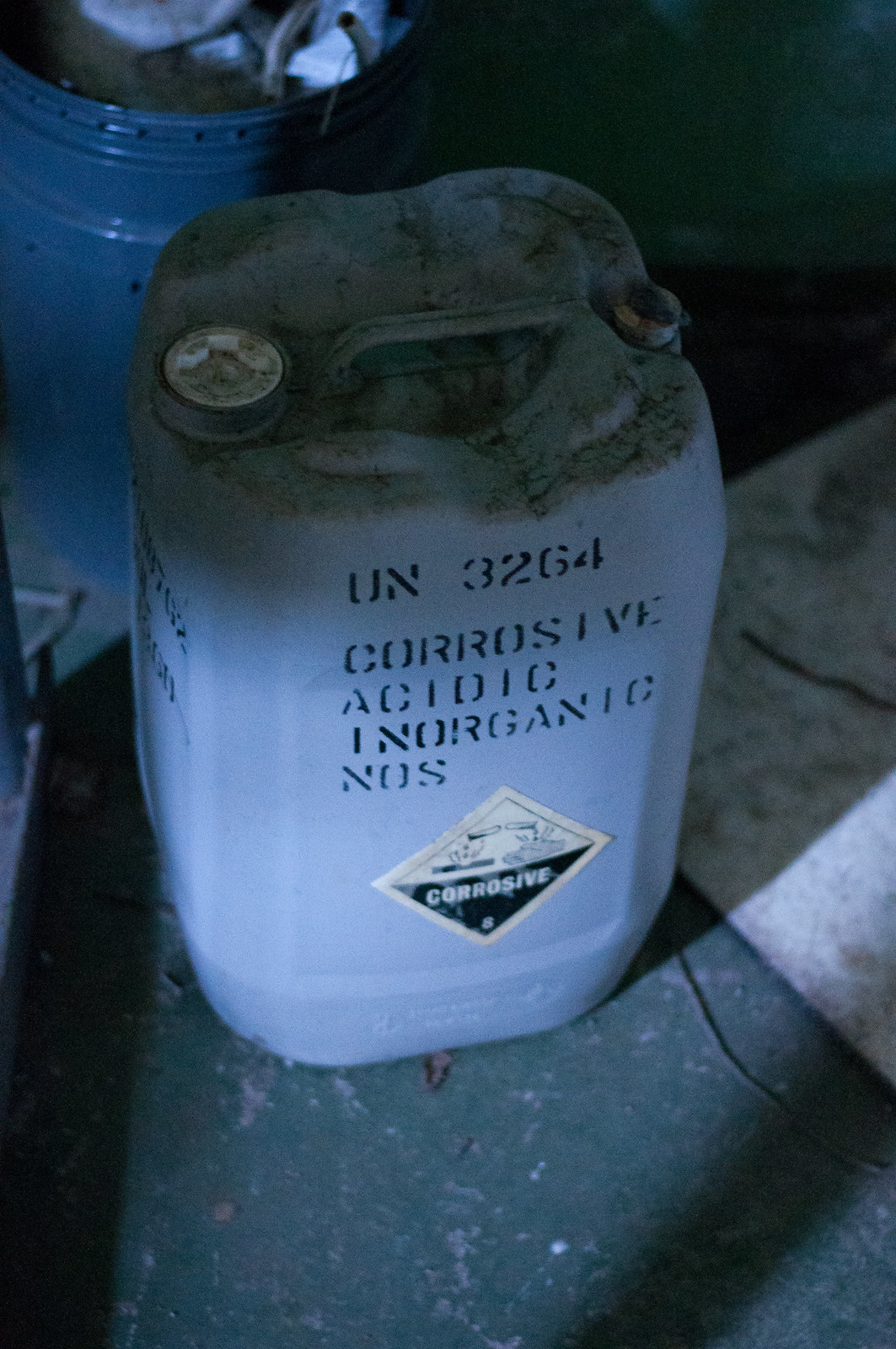The image is a dark, indoor photograph taken in a garage or workshop. The focal point is a light blue or bluish-gray metallic container resembling a gas can, prominently positioned at the center. It features a built-in handle at the top, with two round openings for air and pouring, situated on the left and right sides. The top of the container is dirty and slightly corroded, indicative of prolonged exposure. Written on the front of the can in black lettering are the codes "UN-3264" and "Corrosive, Acidic, Inorganic, NOS," along with a black and white triangular warning sticker indicating "corrosive." Behind this container, there is a blue five-gallon bucket filled with some kind of trash and accompanied by a white towel on the floor beside it. The scene is set against a dark green floor and a gray wall, with very little light entering from the left, creating a dim ambiance.